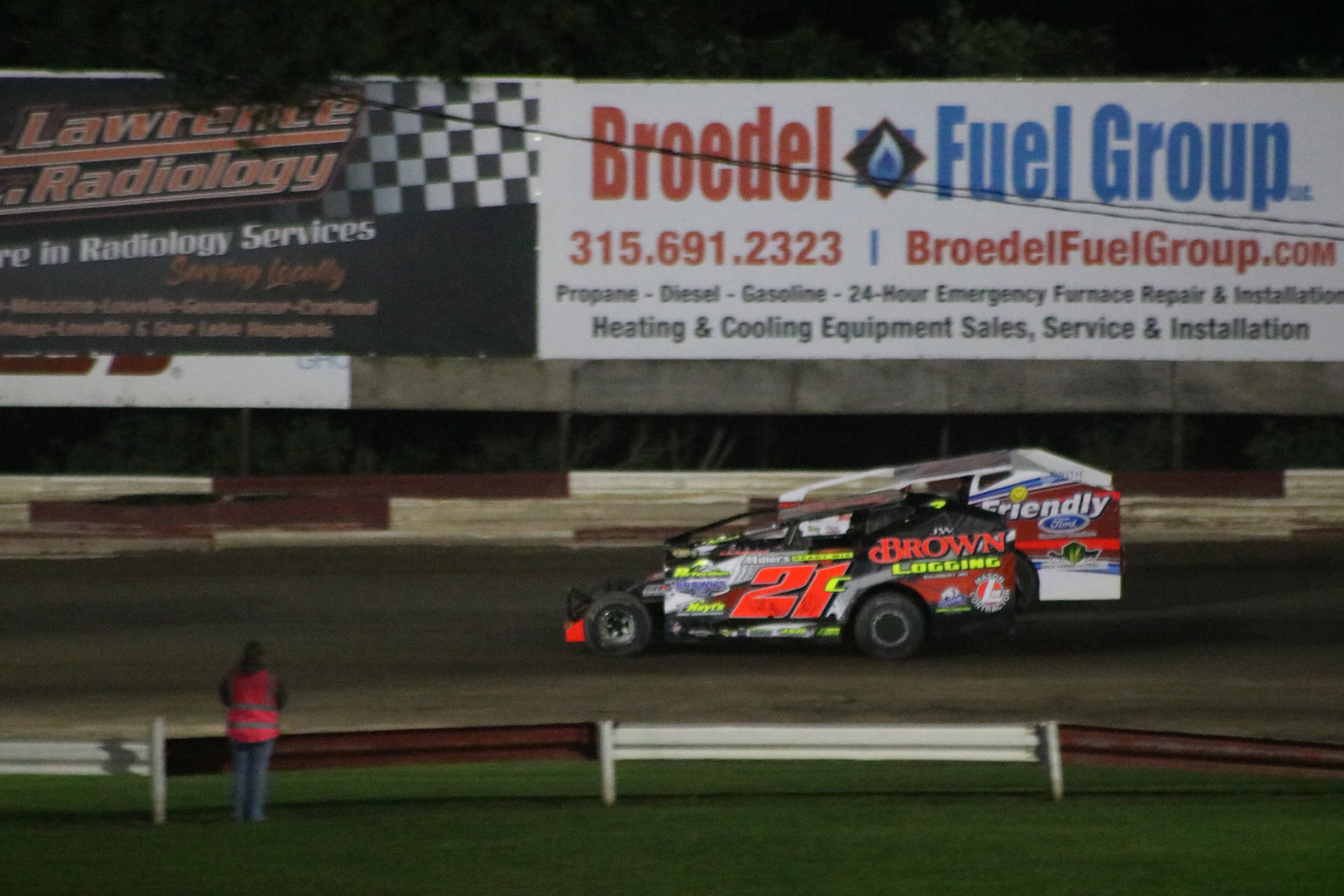The image captures a dynamic moment from a racing rally, prominently featuring a number 21 car as it speeds leftward on the track. The car, adorned with vibrant, multicolored graphics and an orangish-pinkish number on the driver’s door, exudes an air of high-speed excitement. Its design includes a pointed front and a flared back, enhancing its aerodynamic profile. 

In the background, various advertisements span the scene. A notable banner for Brotal Fuel Corp takes center stage, sporting a blue propane flame beside detailed text including a phone number (315-691-2323) and various services such as propane, diesel, gasoline, and 24-hour emergency furnace repair and installation. Additional claims about their heating and cooling equipment sales, service, and installation are also visible. 

To the left, partially cut-off signage promotes Lawrence Radiology Services, although some text remains unreadable as it extends beyond the frame. Beneath these ads, a person clad in a red reflective vest stands watchfully behind a fence, embodying the sense of vigilance and safety typically found at such events.

The scene is captured with a realist photographic style, offering a detailed and immersive visual portrayal of the rally’s intensity and the surrounding environment.